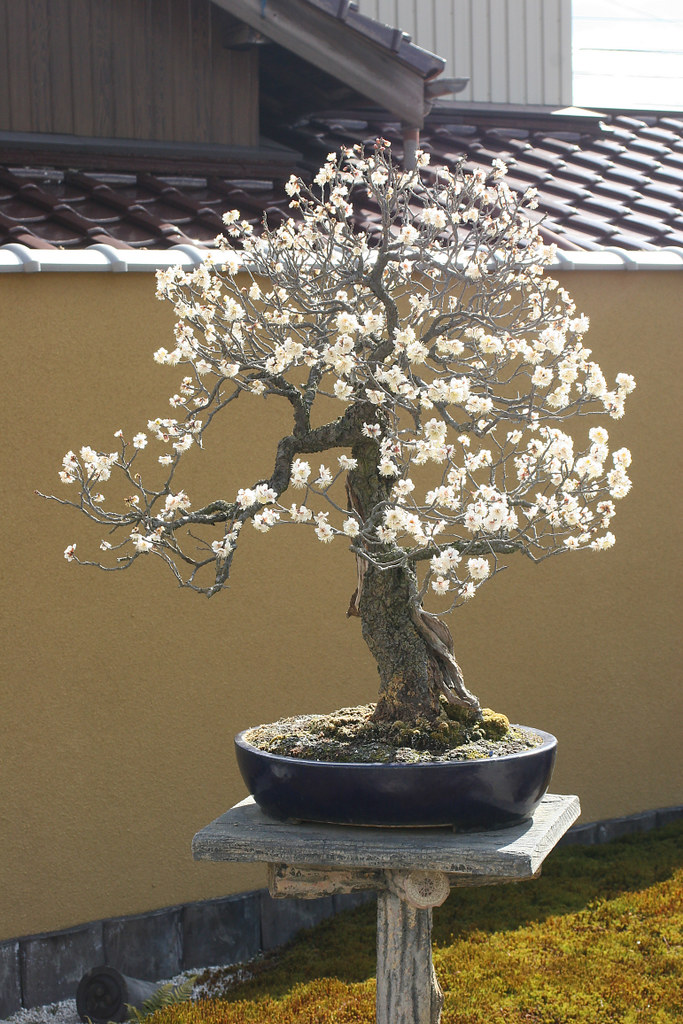In the image, we see the backyard of a home, likely situated in Japan, given the architectural details visible at the top of the photo, such as the distinctive shingle design reminiscent of traditional Japanese architecture. The focus of the scene is a cement post in the foreground. Atop this cement post sits a potted bonsai-like tree. The tree is small but adorned with delicate white flowers. However, some branches appear dry and aged, suggesting that the tree might be in the later stages of its life cycle, potentially causing the white flowers to bloom as a final flourish. The overall scene captures a serene yet somewhat melancholic glimpse of natural beauty intertwined with traditional architectural elements.